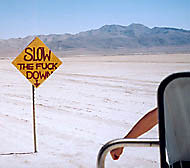In the image, a roadway sign stands prominently against a rugged desert backdrop. The sign, emblazoned with the bold and explicit directive, "Slow the fuck down," features an arrow pointing downward, demanding the attention of any passersby. The terrain appears to be a mix of sandy hues, transitioning from a light, almost white sand in the foreground to a more traditional desert sand color as the landscape stretches towards the horizon. Beyond the sign, majestic mountains rise up, framed by a clear blue sky devoid of any snow, further confirming the desert setting. On the bottom right of the image, the reflecting arm-extension and black trim of a large truck’s mirror come into view. Partially visible within the mirror is a fleeting glimpse of an arm, suggesting a person caught mid-stride behind the vehicle, adding a human element to the stark, solitary scene.